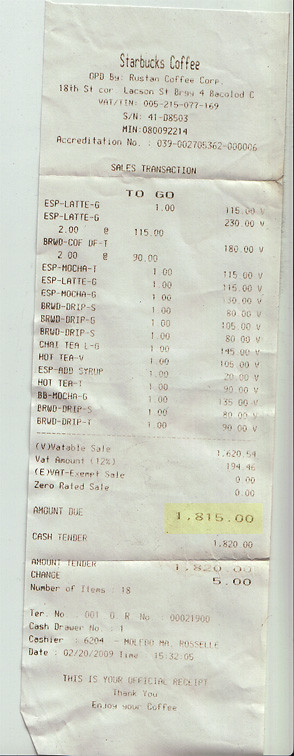This close-up image showcases a slightly worn elongated white receipt against a white tabletop surface. The receipt appears to originate from Starbucks Coffee, evident from the logo and branding at the top. The tabletop underneath is barely visible, with just a narrow sliver of white peeking out. 

From the details on the receipt, it’s clear that the total amount due is $1,815.00, though it appears slightly faded and worn towards the bottom. Additionally, the change amount displayed is $5.00. The receipt lists various items and their corresponding prices; however, these details are also somewhat faded and worn, indicating wear and tear at the lower section. Despite this, the overall layout and format typical of Starbucks receipts remain recognizable.